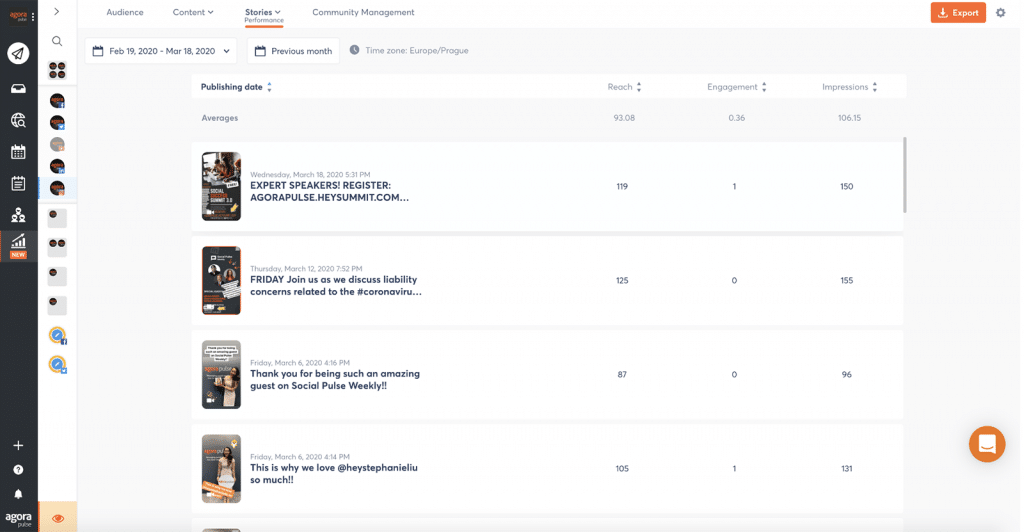This image is a detailed left-to-right horizontal screenshot from a digital platform, viewed either on a computer or a smartphone. The top, left, right, and bottom edges of the screen are bordered by gray lines, with a thick black vertical line running down the left-hand side. At the top of the screen, there are tabs labeled "Audience," "Content," "Stories," and "Performance," the latter highlighted by a small orange line underneath it. To the far right, there is an orange rectangle button labeled "Export" beside a settings icon.

Along the thick black line on the left are several clickable icons: a calendar, an airplane symbol, a group of people icon, a plus sign, a question mark, and a bell. Adjacent to these, on a white strip, are additional clickable icons such as a magnifying glass, a four-circle grid, and several circular icons.

On the right-hand section of the screen, there is a date range displayed: "February 19, 2020 to March 18, 2020." Below this, options like "Previous Month," "Time Zone," "Publishing Date," "Reach," "Engagement," and "Impressions" are listed. In the central part of the image, it mentions an event titled "Expert Speaker Register," associated with the platform "Agorapulse" hosted on "heysummit.com." There's an announcement for a Friday event discussing liability concerns, a thank-you note to a guest on "Social Pulse Weekly," and icons representing reach, engagement, and impressions, alongside detailed metrics for each.